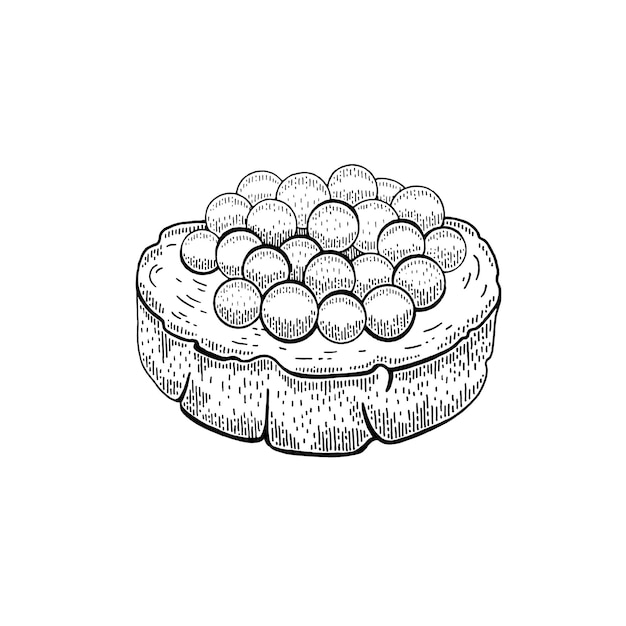This black and white drawing, rendered in a simple line style, depicts a circular piece of wood or large slice of bread, intricately detailed with hundreds of small lines that create texture. Atop this base is a mound of round objects that resemble beads, pearls, or caviar eggs. These balls vary in size, adding to the textural complexity. Some interpretations describe it as marbles piled on a tree stump, while others see it as a lavish caviar sandwich with the eggs scattered on a slice of bread. The drawing's ambiguity and detailed line work invite multiple perspectives, reminiscent of both natural and crafted compositions.